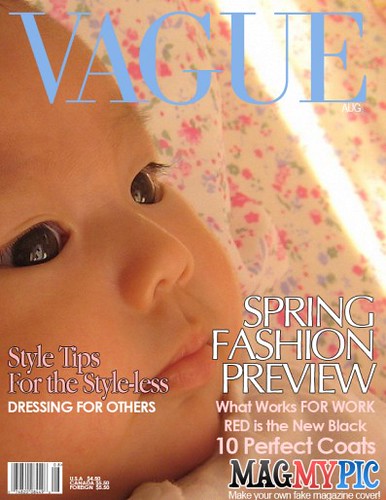This image features a satirical magazine cover titled "Vague" mimicking the iconic Vogue font and style. Centered on the cover is an adorable baby with no hair, seemingly gazing at something off-frame. On the lower left side, an ISBN code adds to the faux authenticity. Surrounding the baby’s face, the cover features multiple headlines such as "Spring Fashion Preview," "What Works for Work," "Red is the New Black," "Ten Perfect Coats," and a colorful watermark stating "Mag My Pick," suggesting the image could be used to create custom fake magazine covers. Printed directly on the baby’s cheek are the phrases "Style Tips for the Stylists" and "Dressing for Others." The overall design aims to humorously emulate an old-school magazine aesthetic.